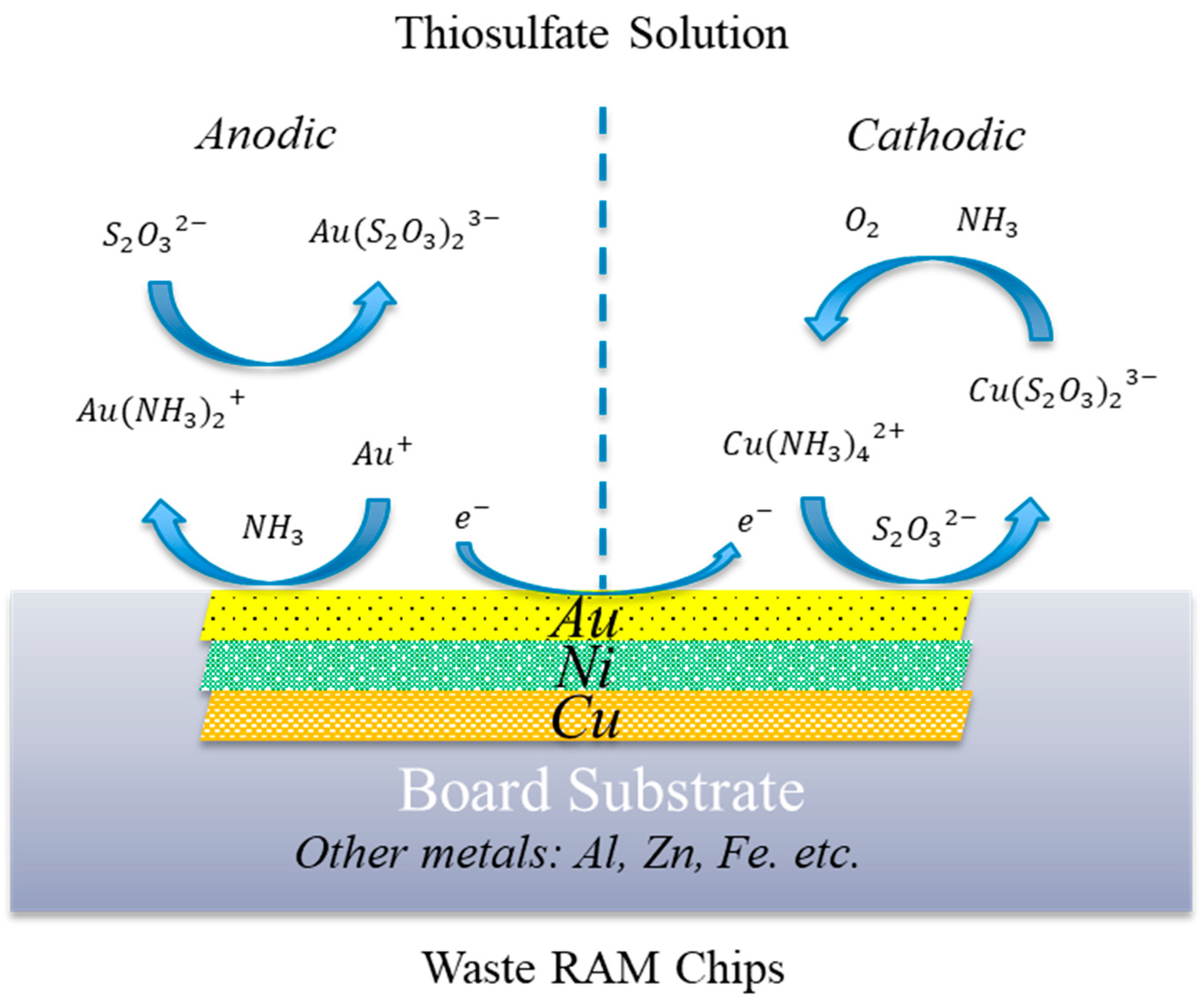This intricate diagram, prominently titled "Thiosulfate Solution" at the top in large black letters, is divided into two sections by a central blue dotted line. The left section is labeled "Anodic" and the right section "Cathodic". Each side features detailed chemical processes depicted with blue arrows connecting various molecular formulas. In the anodic section, compounds such as \( S_{2}O_{3}^{2-} \) and \( AU(S_{2}O_{3})_{2}^{3-} \) are illustrated, with arrows indicating chemical reactions. The cathodic side mirrors this setup with its own set of chemical reactions and blue arrows denoting direction. Below these molecular illustrations, a bright bar of yellow, green, and beige rectangles displays the letters \( Au \) (gold), \( Ni \) (nickel), and \( Cu \) (copper). Further down, the text mentions "board substrate," "other metals" including \( Al \) (aluminum), \( Zn \) (zinc), \( Fe \) (iron), and "etc.," culminating with "waste RAM chips" at the very bottom.